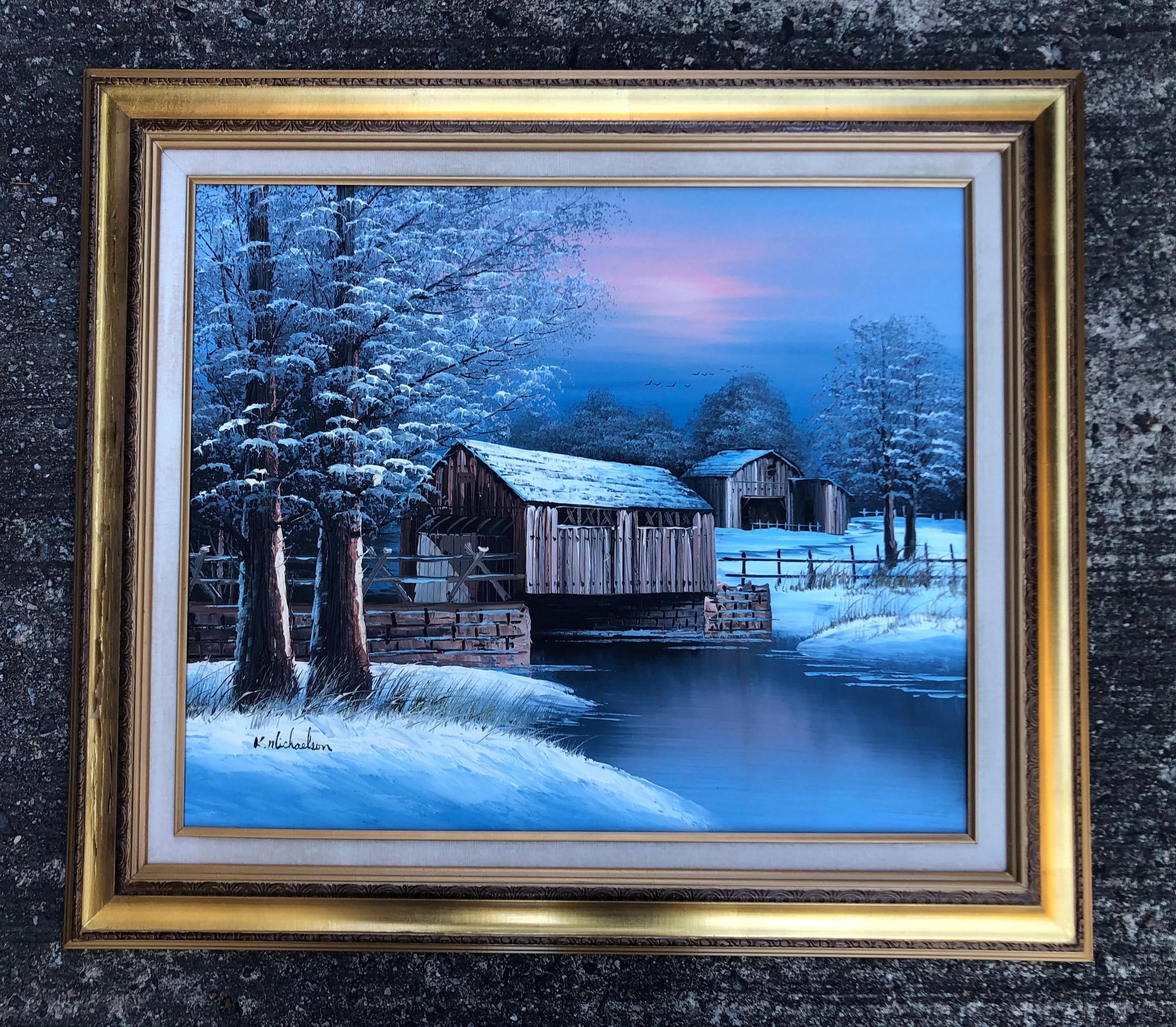This image features a framed piece of wall art set against a textured, dark black and charcoal wall. The frame is a brilliant gold with a beveled edge, comprising multiple intricate layers: an outer wood-looking edge, an ornate carved gold inner frame, and an additional small white border with another gold inner lining. The artwork within the frame is an oil painting of a winter landscape. It captures a serene scene of a wooden barn and a shed with snow-covered roofs in the background. To the left of the painting are two snow-laden trees, their branches heavy with white. In the foreground, a stone bridge with a wooden covering spans a dark blue river, its roof glistening with snow. The sky features hues of light blue and pink, and the artist's name, appearing as K-M-L-I-C-H-A-E-T-S-O-N, is signed in the lower left-hand corner.